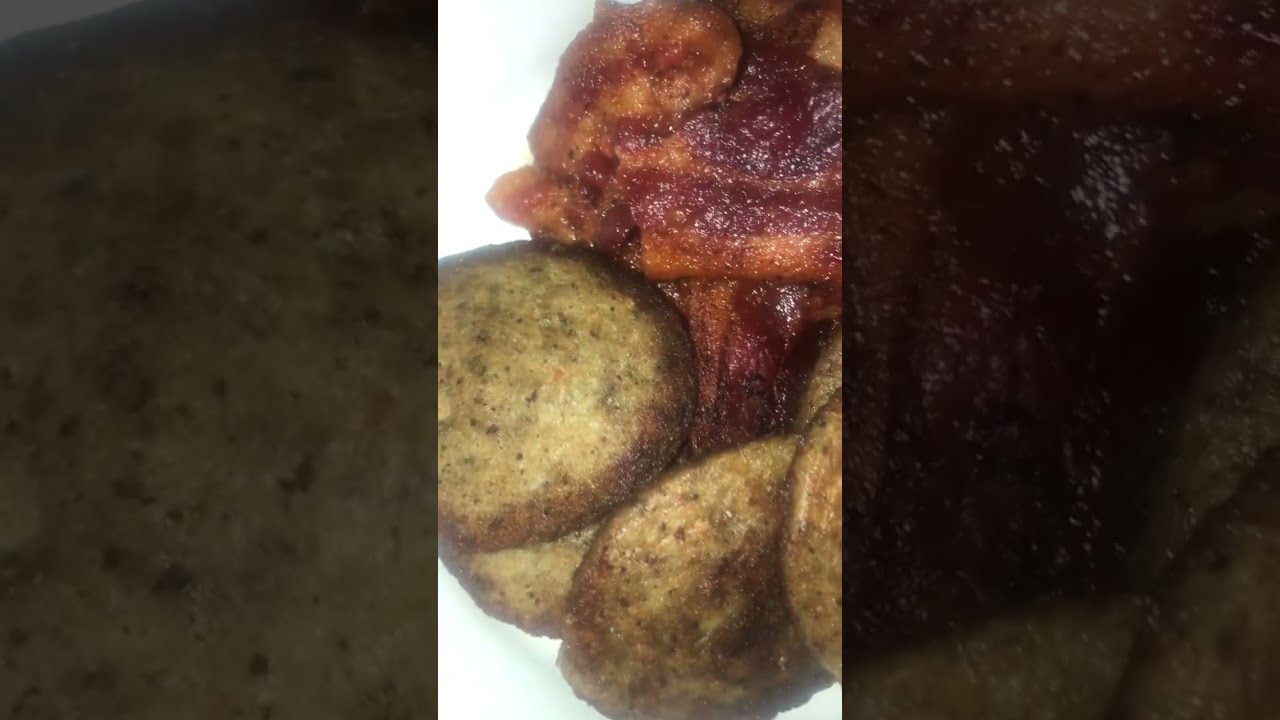The image is a close-up culinary photograph featuring a detailed arrangement of various food items. In the center of the image, there is a stack of light green cookies with brown edges, dotted with green and black speckles. These cookies are piled up on top of each other, partially obscuring a shiny, heavily glazed muffin with a dark amber exterior, reminiscent of syrup rolling down its surface and an orange hue in the middle. The background is a stark white, with close-up trims on the left and right sides showing reflective glimpses of the muffin's glaze. 

In addition to the cookies and muffin, there are slices of what seem to be home fries or possibly mushroom caps, characterized by dark brown edges and lighter brown centers, some stacked and others standing on their sides. On the top portion of the plate, there is an arrangement of crispy, well-cooked bacon, forming an X shape. Below the bacon, light brown sausage patties with green seasoning and searing marks are visible, adding to the rich textures and colors. The entire image is set against a white plate, which highlights the intricate details and contrasts of the food items.